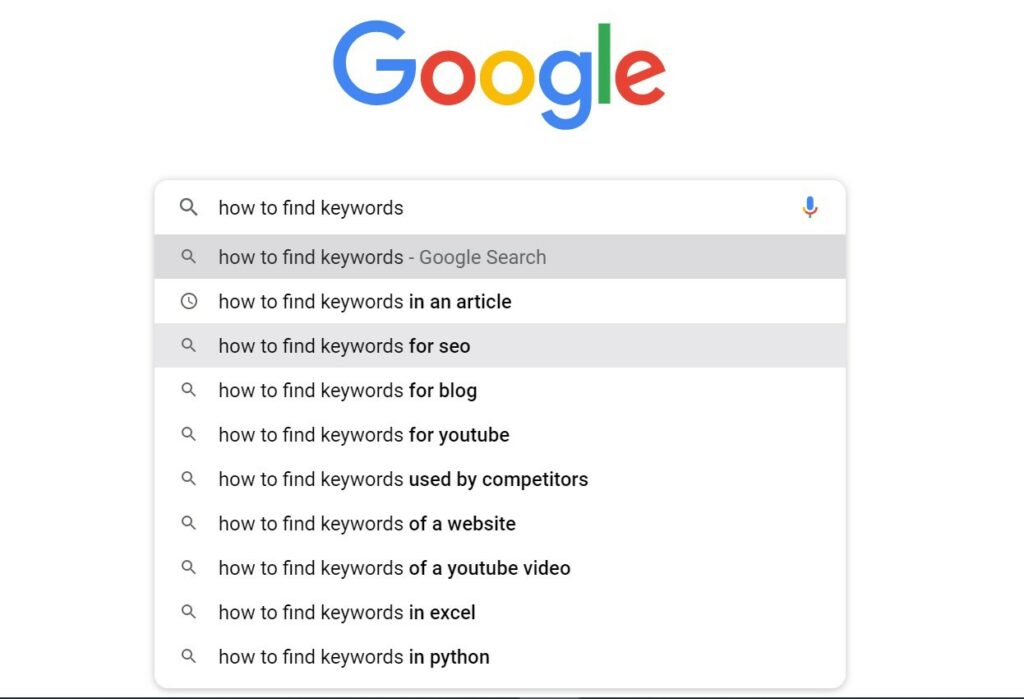Screenshot of a Google Search Page Before Query Submission

In this image, we see a Google search page captured just before a search is initiated. Prominently featured at the top is the iconic Google logo, beneath which lies the familiar search bar. Within the search bar, the phrase "how to find keywords" has been typed. Adjacent to the search query on the right is the search icon, and further to the right is the voice search icon.

Directly below the search bar, suggestions related to the typed query appear. "How to find keywords in an article" is marked as previously searched, while other suggestions including "how to find keywords for SEO," "how to find keywords for blog," "how to find keywords for YouTube," "how to find keywords used by competitors," "how to find keywords of a website," "how to find keywords of a YouTube video," "how to find keywords in Excel," and "how to find keywords in Python" are displayed but not previously searched. These suggestions are encased within a rounded gray box.

Just beneath this suggestion box, a thin black line denotes the end of the page. The rest of the page is minimally designed, with only the white background visible beyond the search suggestions and Google logo. This clean and simple layout emphasizes the search functionality of the Google homepage.